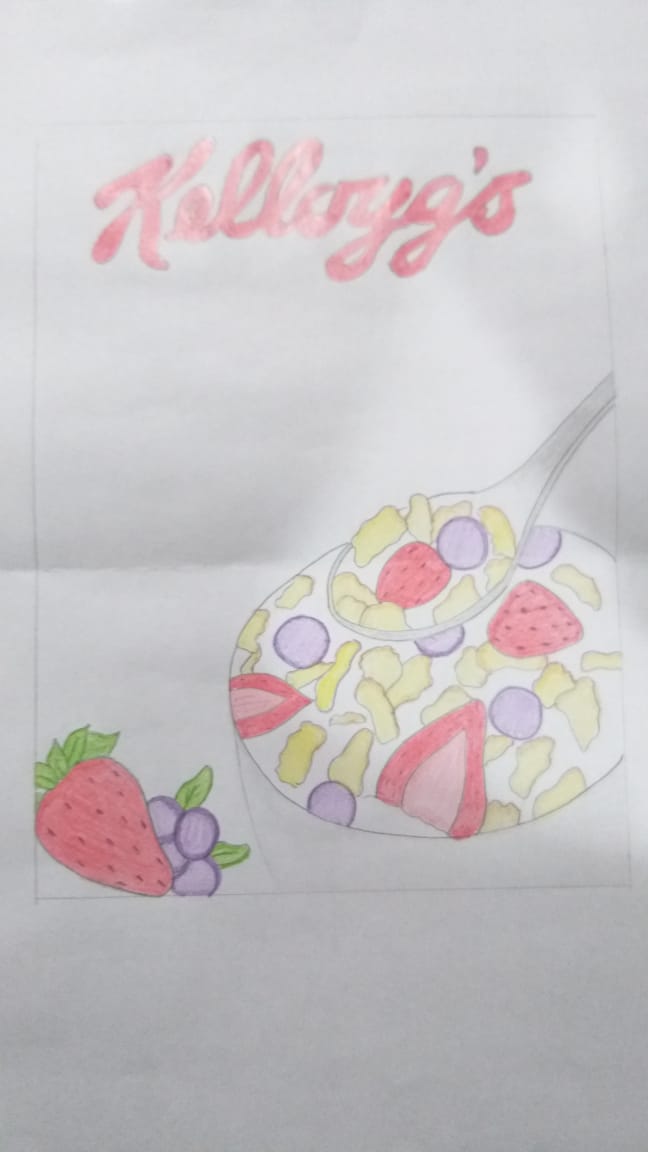This is a detailed drawing on a white piece of paper that resembles a cereal box design. At the top, in red bubble letters, is the Kellogg's logo, spelled K-E-L-L-O-G-G-apostrophe-S. The logo is intricately drawn in a cursive style. Beneath the logo, across the middle section, is a bowl brimming with cereal, depicted with various colors. The bowl contains milk, cereal pieces, and slices of strawberries and blueberries. A silver spoon is visible from the edge of the drawing, holding milk, cereal pieces, a strawberry half, and a blueberry. In the bottom left corner of the drawing, there is a detailed depiction of a whole strawberry with black seeds and a green stem, accompanied by a cluster of shaded blueberries and green leaves. The colors used in the drawing include red, green, purple, yellow, pink, and black, which stand out vividly against the white background. The image is framed by a thin black rectangular border, drawn in a portrait orientation. This artwork remains unsigned by the artist.